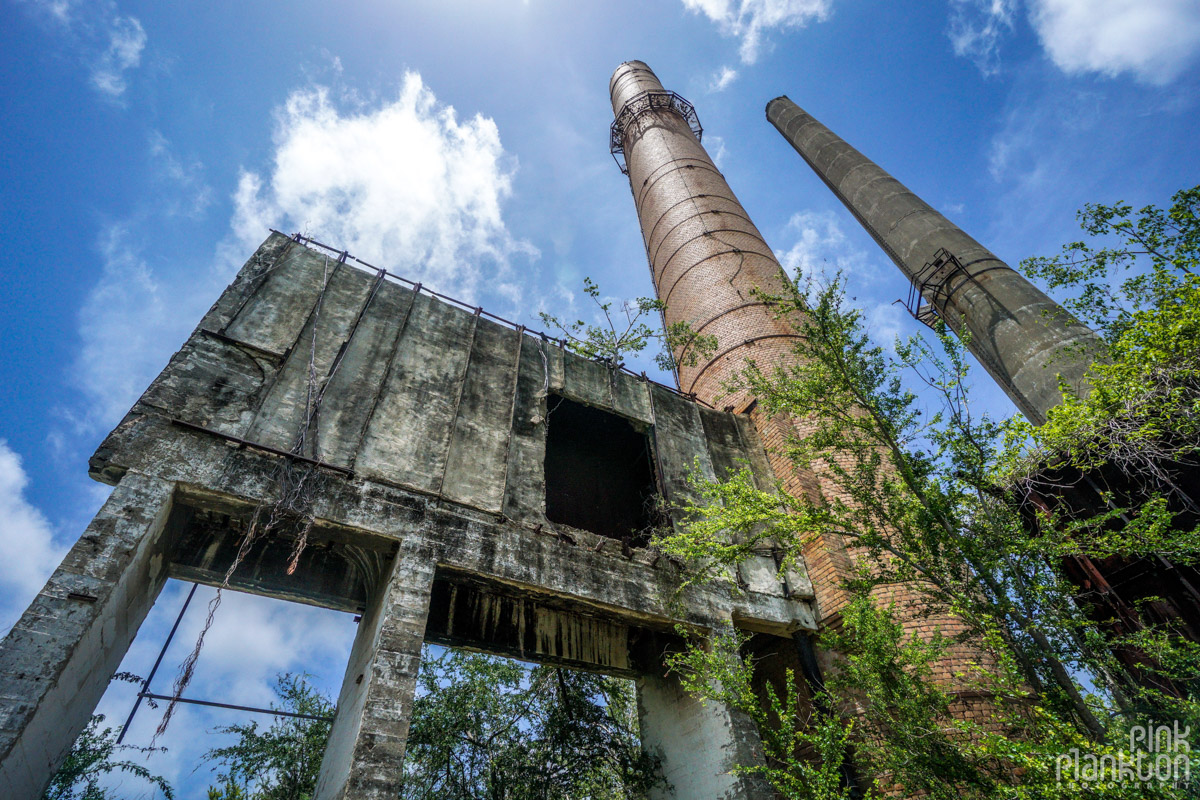This color photograph captures an outdoor daytime scene from ground level, looking upward at the dilapidated remnants of an abandoned factory. Dominating the center of the image is a tall, red brick smokestack, with a metal walkway encircling its upper section and wires running down its side. To its right stands a shorter, dark gray concrete smokestack with a ladder extending from the bottom to the top. Adjacent to these smokestacks is a large, dirty, and discolored concrete wall, with significant portions missing, revealing glimpses of bushes and the blue sky beyond. The old factory wall also has open, rectangular spaces where loading bays and doors once were, now edged with black soot. The area is heavily overgrown, with vegetation, trees, bushes, and vines encroaching upon and intertwining with the decaying structures. The sky overhead is a vibrant blue, dotted with wispy white clouds, and the sun casts a soft, glowing light just out of frame, illuminating the entire scene.